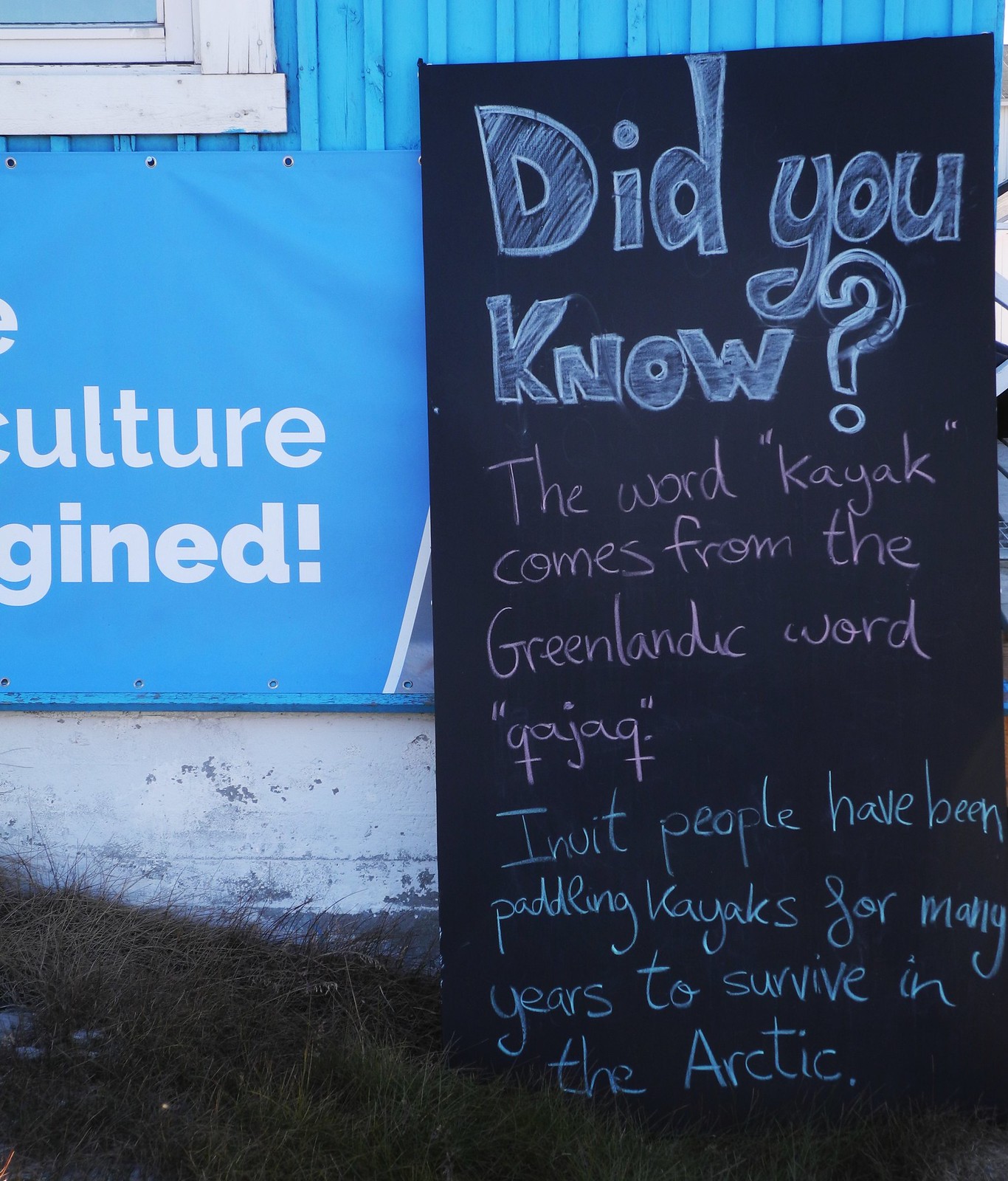This image features a tall, rectangular black chalkboard propped against the wall of a blue and white building. At the top of the blackboard, in white chalk, is written "Did you know?" with a question mark. Below it, in pink chalk, it states, "The word kayak comes from the Greenlandic word, 'kajak'." Further down, in blue chalk, it reads, "Inuit people have been paddling kayaks for many years to survive in the Arctic." The chalkboard is resting on grass, and you can see part of a white-trimmed window in the upper left corner of the image. The building has blue side panels and a barely readable banner at the bottom, with white concrete visible at the base with gray splatterings. The whole scene is slightly inclined, with the grass highest on the left side and sloping downward to the right.